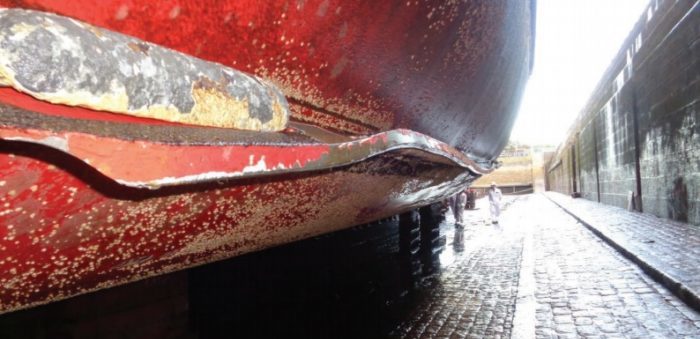The photograph captures a bright sunny day on a city cobblestone street, bordered by a concrete wall on the right. Dominating the scene is an enormous red object, extending from the bottom left corner to three-quarters up the page. The object is characterized by a worn, scraped-up surface with white and brown speckled patches, likely indicating rust and oxidation. A heavily rusted red metal band runs diagonally from the left middle, down the figure, to the right end. Toward the bottom right, a black support structure is visible. The stone street showcases individual cobblestones, highlighting the rough and uneven texture, while the brick walkway adds to the urban atmosphere. In the mid-right section, two small figures in light-colored suits (appearing to be male) provide a sense of scale, emphasizing the object's immense size. Behind them stands a beige-colored building, enhancing the historic and weathered look of the scene.